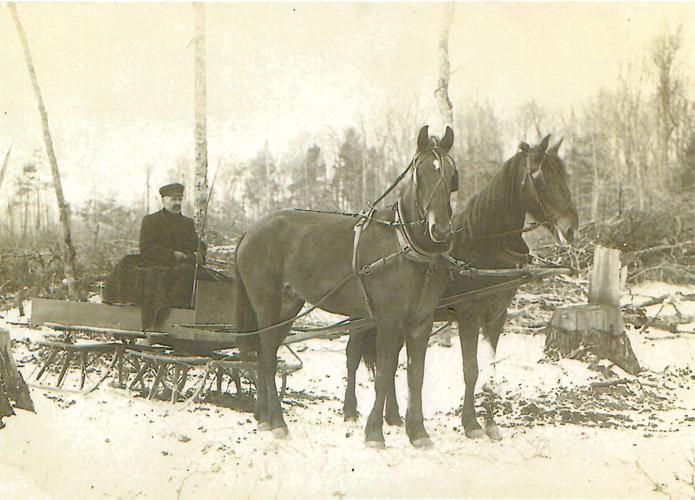In this aged, black-and-white (almost sepia-toned) photograph, a man in a heavy black coat and hat sits in a makeshift wooden horse-drawn cart. The cart, equipped with skis for navigating through snow, is pulled by two bridled black horses that stand side by side, facing to the right. The man holds the reins firmly, a blanket draped over his lap. The ground is covered in a light layer of snow, and scattered around are remnants of a forest— a mixture of standing, fallen, and chopped down trees, with noticeable stumps. The scene captures a side view of the wagon and horses, set against the stark backdrop of a partly decimated woodland area. Amidst the trees, some larger trunks stretch skyward, untouched by the apparent destruction that has felled their companions.